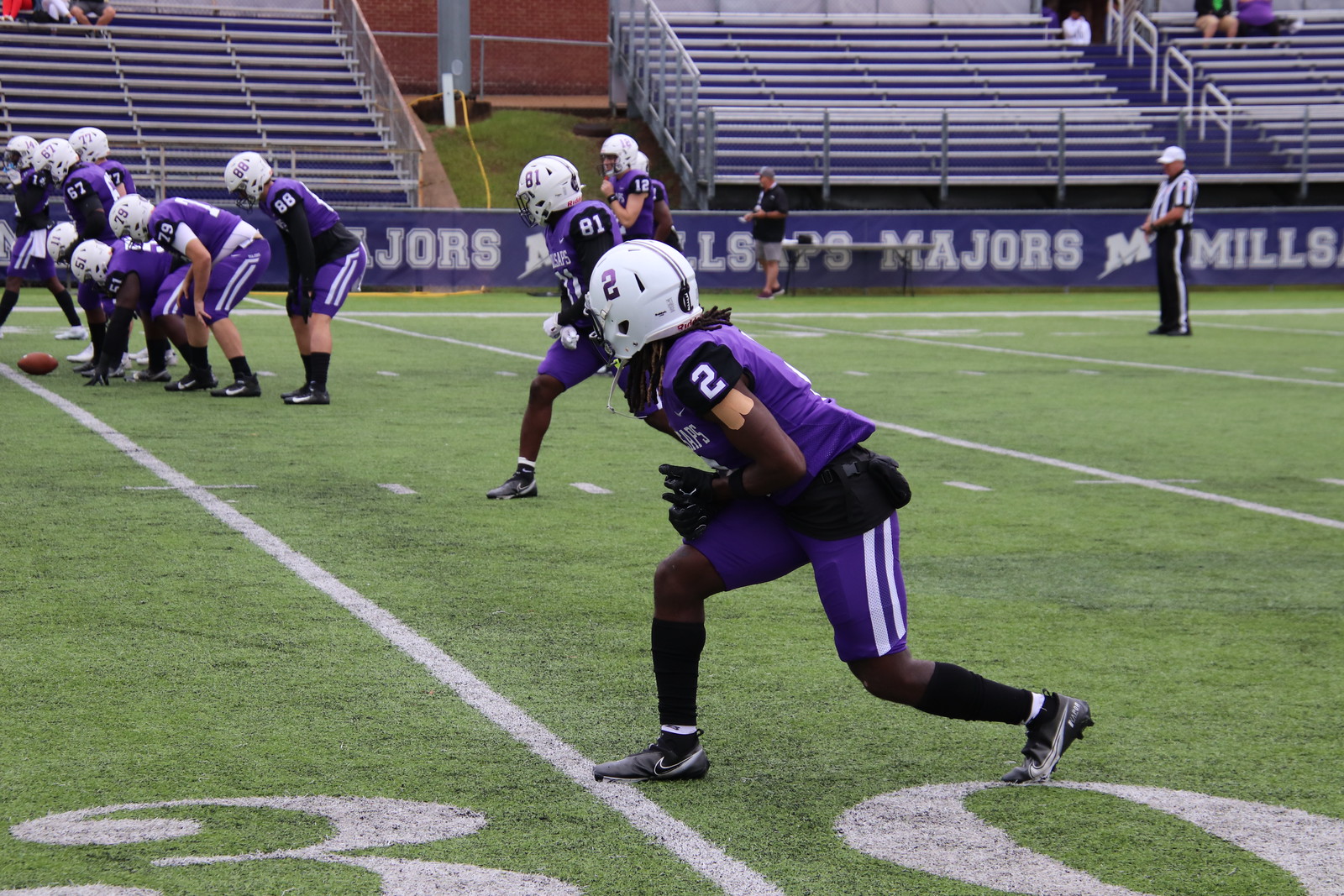The photograph captures an American football game in progress. The offensive team, distinguishable by their purple uniforms and white helmets, is lining up for a play. The ball is positioned on the 30-yard line, clearly marked by a large white number "30" on the grass. In the foreground, closest to the camera, player number two is seen lining up wide, poised with his right toe on the 30-yard line and his left leg behind him. Further up the field, the center is about to hike the ball to the quarterback, who stands around the 35-yard line.

In the background, we can see almost empty bleachers with a fence bearing the words "majors" and "Mills." A referee in black and white stripes, stationed in the upper right-hand corner, watches the developing play. Along the bottom part of the field near the barrier, a person dressed in black can be seen walking or spectating. The stands are sparsely populated, with only one or two spectators visible. The green field is evenly lined, adding structure to the scene, and the overall setting includes additional players in various positions and an assortment of stadium structures such as rafters and a building visible from the center and upper left part of the image.